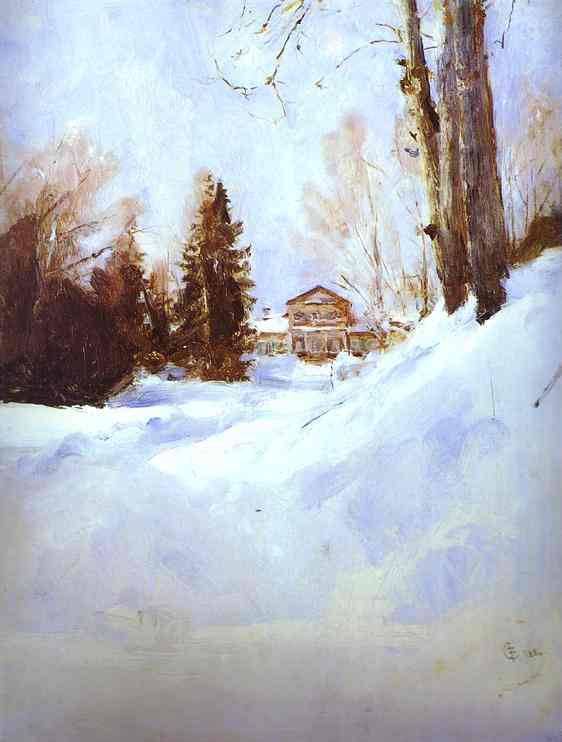The painting is an outdoor winter scene, beautifully captured in oils, with a snow-covered ground that occupies nearly half the image. The snow slopes gently from right to left, creating a subtle gradient of white and pale blue shades, with a hint of brown near the bottom edge. On the right side, a few tall brown tree trunks rise with bare branches extending toward the top of the painting. The left side features thick, bushy brown brambles and pine trees, which are also rendered in brown rather than green.

In the background, a prominent two-story cabin or large house, with a slanted roof painted in a blend of brown and white, stands amidst the trees. Additional houses are nestled below it. The sky above is a light blue, interspersed with shades of gray, closely matching the hue of the snow-covered landscape. The painting, which is in portrait orientation, bears a hint of the artist's signature in a different color in the bottom right-hand corner, although it is not clearly legible. Overall, the composition harmonizes the white and blue tones of the sky and snow with the brown elements of the trees and structures, creating a serene and cohesive winter scene.